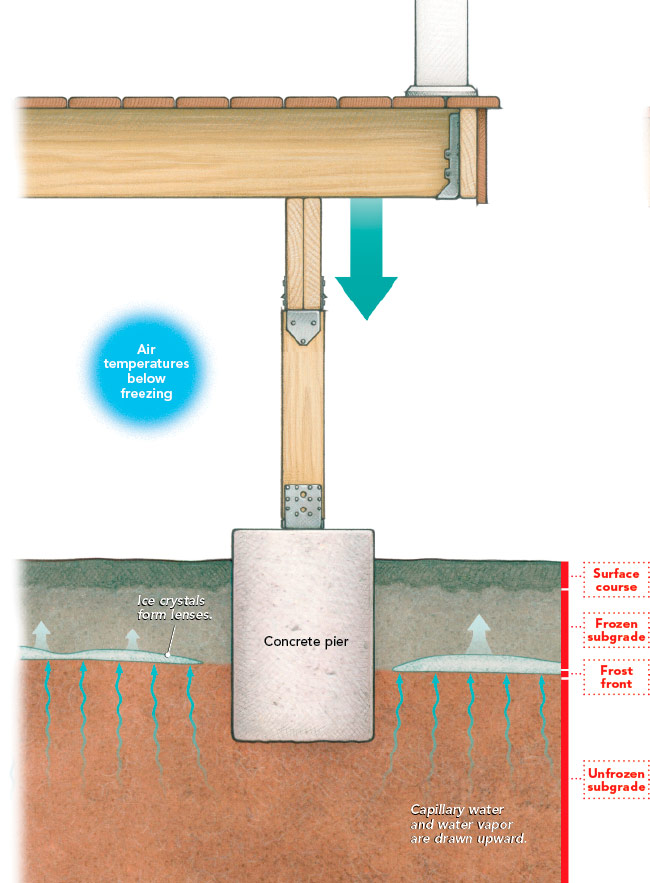This is a detailed, colored textbook-like diagram illustrating the insertion of a post into the ground for a porch. The background is white, and at the base, there is a brown dirt layer with wiggly blue arrows pointing upward, five on each side. Text within this layer reads, "Capillary water and water vapor are drawn upwards." Above the dirt layer, a sequence of labeled layers is displayed: first, a gray layer called "frozen subgrade," followed by a green layer indicating the grass surface. 

Emerging from the dirt, a large light gray cylindrical structure labeled "concrete pier" stretches upward through these layers. At the top of the pier is a wooden post secured with metal hinges, supporting a small deck structure, a segment of which is visible along with part of the flooring.

On the right side, additional labels delineate the different earth strata: "Surface course," "frozen subgrade," "frost front," and "unfrozen subgrade," each enclosed within dotted red boxes. At the top of the deck, a blue arrow points downward, and text reading "Air temperatures below freezing" is enclosed in a blue circle in the top left corner.